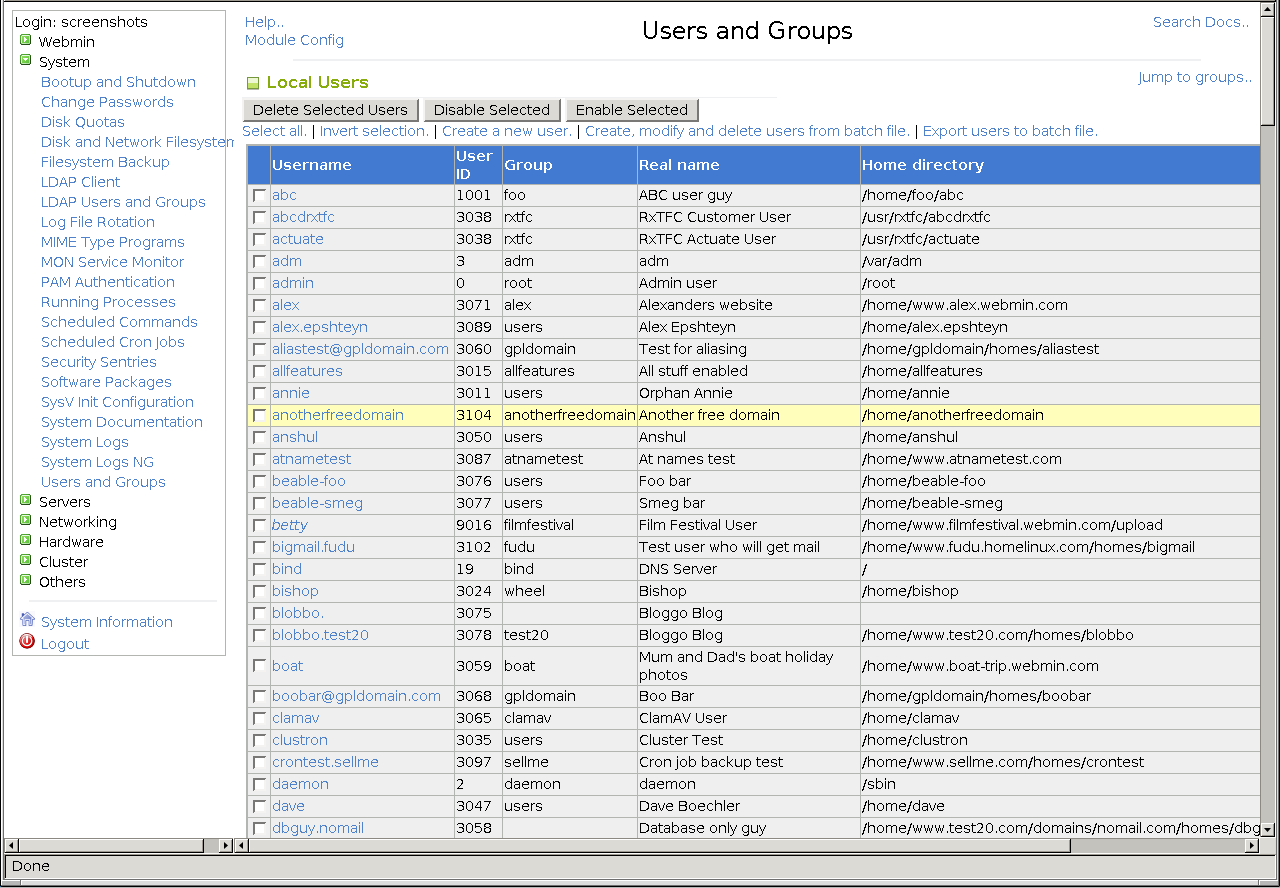Screen capture showing the backend of an admin area for a website, encapsulated within a light gray border. A vertical gray scroll bar is positioned on the right-hand edge, allowing navigation through the content.

In the top-left corner, the bolded black text reads "Login Screenshots." Beneath this, in black, are the headings "Webmin" and "System." Adjacent to these headings is a green square with a white right-arrow, resembling a play button.

Below, a series of extensive blue labels pertain to various administrative functions such as Boot Up and Shutdown, Change Passwords, Disk Quotas, LDAP Client, LDAP Users and Groups, Log File, Security Settings, Software Packages. Toward the bottom, bolder black labels accompanied by a green button with a white right-arrow include categories like Servers, Networking, Hardware, Cluster, and Others.

Further down, a blue home icon sits to the left of the text "System Information," and at the very bottom, a red turn-off button similar to a Windows shutdown icon is present with the blue text "Log Out" nearby.

The right-hand side features a gray background hosting three columns with approximately 30 to 40 rows. In the top-left, green text reads "Local Users," and centered at the top, bolded black text announces "Users and Groups." Below this header, three rectangular gray buttons with black lettering are labeled "Delete Selected User," "Disable Selected," and "Enable Selected."

A series of blue labels underneath includes options such as "Select All," "Invert Selection," "Create a New User," "Create, Modify and Delete Users from Batch File," and "Export Users to Batch File." A horizontal turquoise blue bar with white lettering identifies the columns from left to right as Username, User ID, Group, Real Name, and Home Directory.

The table beneath these headings details user information, each row containing corresponding data under the specified columns. Accompanying these entries, there are white active checkboxes, none of which are currently checked.